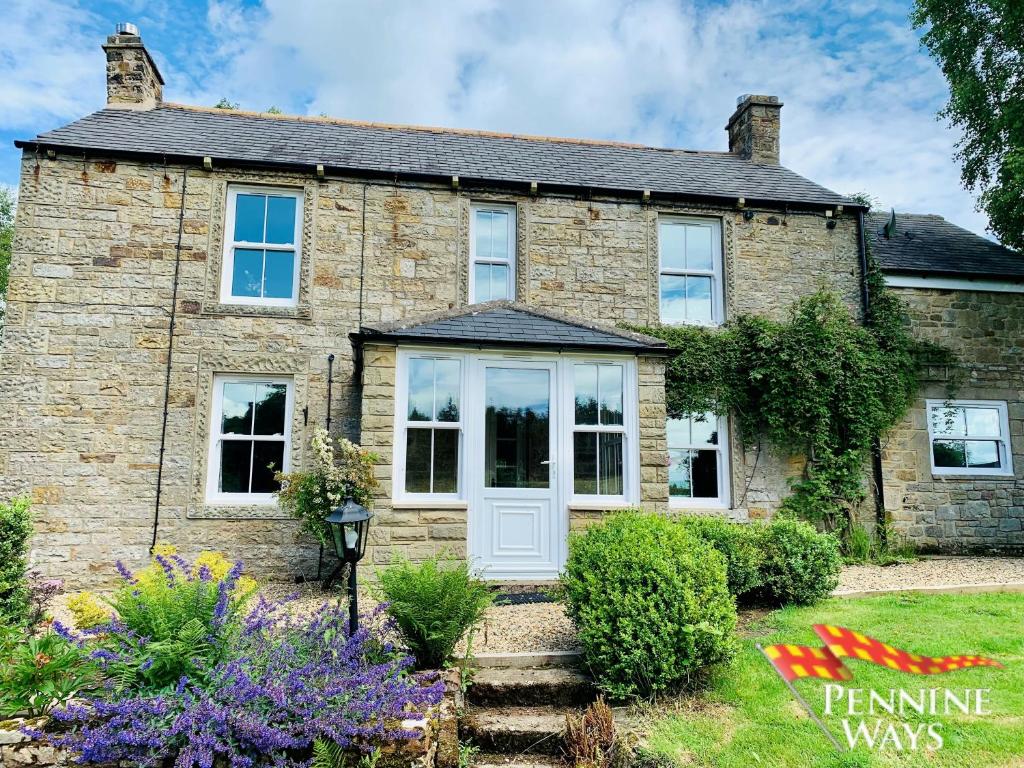This image depicts the back of a beautiful, large, two-story house made of light brown brick, reminiscent of an old-style countryside home in the UK. The house features a total of five vertical rectangular windows: three on the top floor and two on the bottom, all framed in white. The center of the house boasts a white door flanked by two windows on each side. On the far right, there's a small window that seems to belong to an attached section of the house, possibly a garage. Two white-trimmed chimneys rise from either side of the roof. The backyard is adorned with flowers, bushes, and patches of green grass, alongside a bush of lavender that adds a touch of purple. Concrete steps lead up to the back porch, which has two small stairs and is surrounded by tiny rocks. The overall setting is picturesque with a beautiful blue sky filled with white clouds overhead. At the bottom right corner of the image is an emblem of a red flag with yellow squares or polka dots, displaying the text "Pennine Ways" in white.